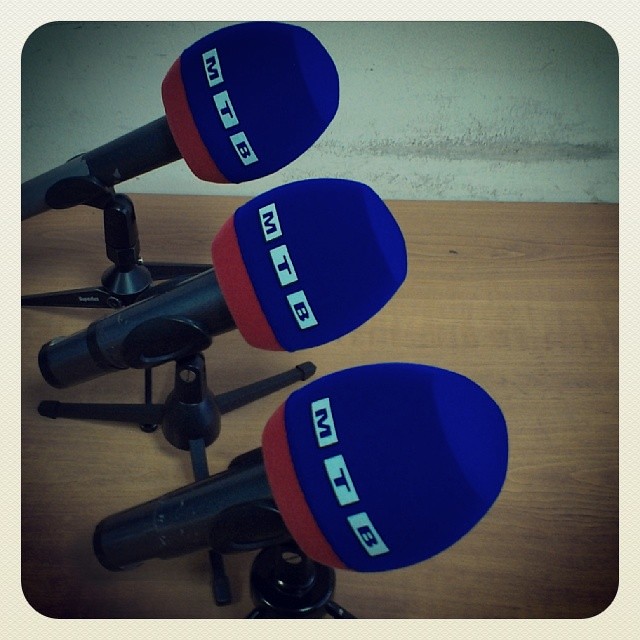This square photograph features three small desk microphones arranged in a vertical line atop a light brown wooden surface, with a smooth texture. Each microphone is on a short black tripod stand and oriented toward the right side of the frame. The microphones have a distinctive design with bright blue foam covers, accented by a red band at the bottom. In the center of each cover, white rectangular boxes with the letters "MTB" are prominently displayed. The background appears to be a white stone or concrete wall, adding to the image's textural contrast. The photo has a subtle patterned border with a diamond and dot motif and features curved edges that soften its square shape. An additional Instagram-like filter enhances the high contrast, making the edges dark and the center brighter, creating a focal light effect on the microphones.